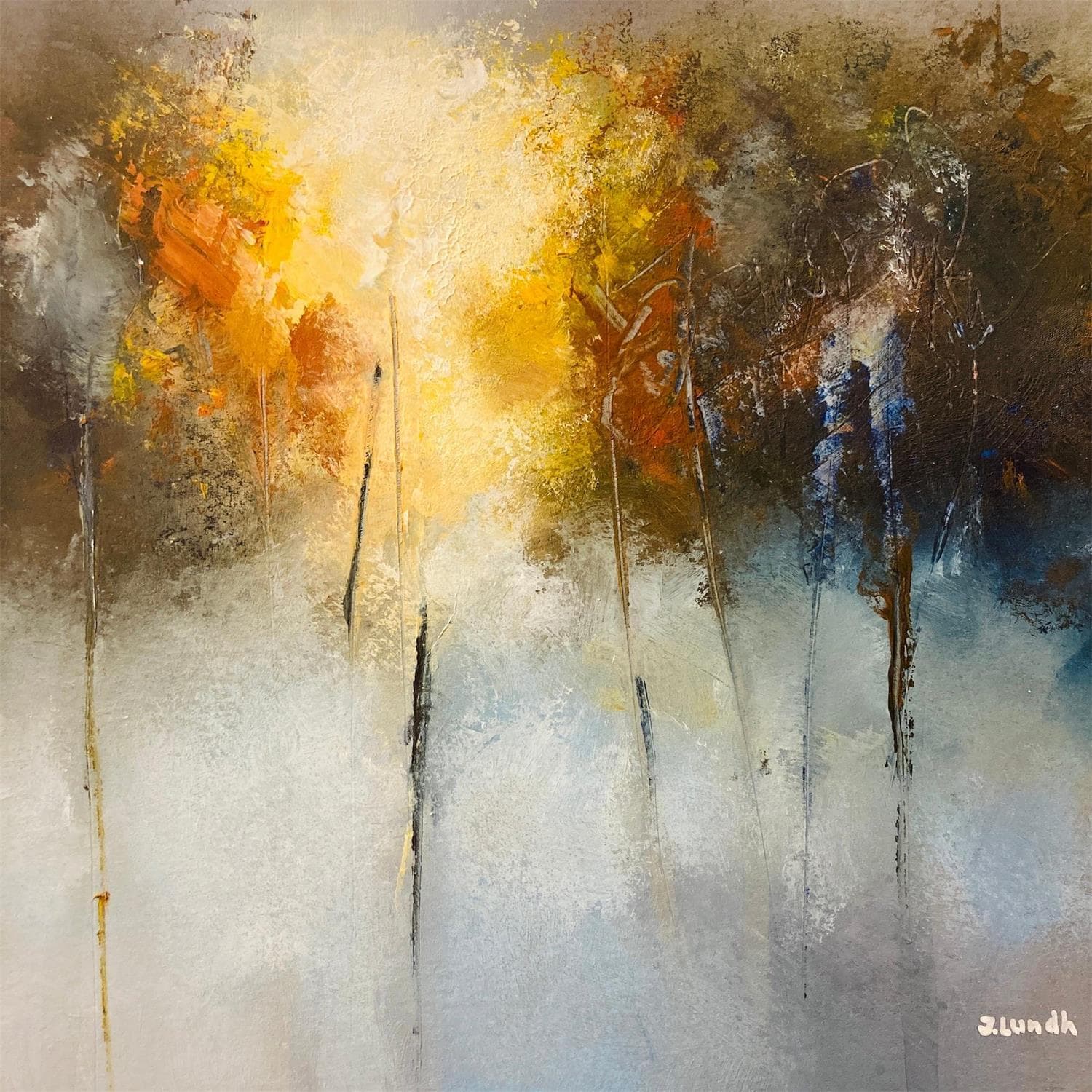This detailed acrylic painting presents a textured, abstract scene dominated by an explosive and dramatic blend of colors. In the lower right corner, the signature of the artist, J. Lundh, can be observed. The bottom half emerges in a foggy white and blue-gray tone, which transitions into tall, slender forms resembling twigs or tall skinny trees shooting upwards. These pierce into the upper half, which bursts with chaotic and violent brush strokes of red, yellow, and brownish green, creating an impression of an explosion. Patches of green and white are scattered throughout, suggesting a resemblance to trees or foliage. Amidst this tumultuous scene, a small faded figure painted in blue can be faintly seen on the right side, adding an enigmatic and ghostly element to the scene. The painting conveys a sense of both energetic eruption and ethereal tranquility, with its cloudy sky and stark contrasts in color and texture.